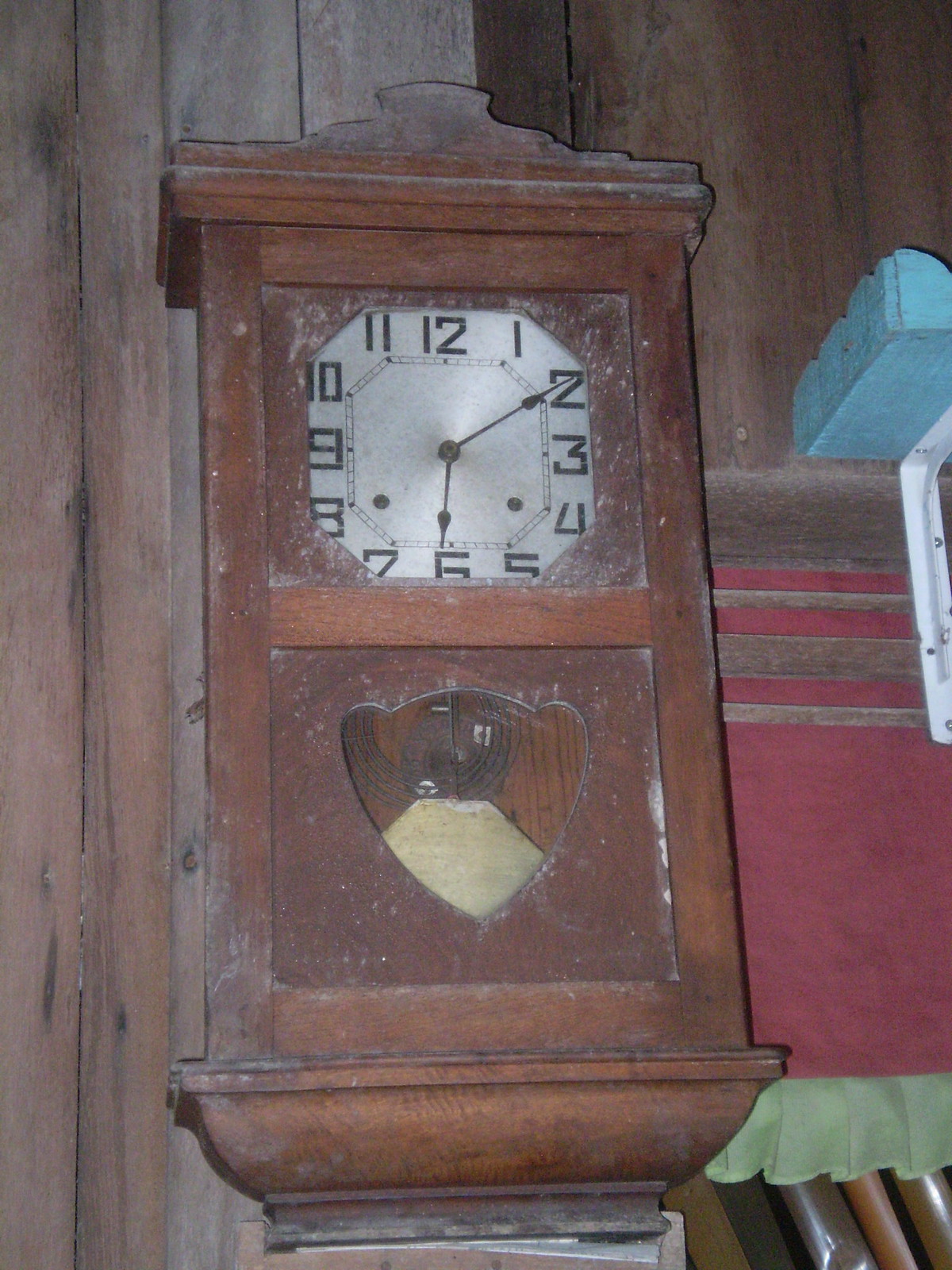The image depicts an antique wooden clock mounted on a wooden wall, covered in a thin layer of white dust that gives it a weathered appearance. The clock face is white with bold black numbering and black hands, displaying the time as 6:10. The numbering is arranged inside a subtly octagonal frame. Notably, the clock has two small rivets situated at the bottom left and bottom right near the center. Below the clock face, visible through a somewhat heart-shaped window, is a bell surrounded by what appears to be red fabric with a yellow ruffle. The overall structure is crafted from brown wood, enhancing its vintage charm.